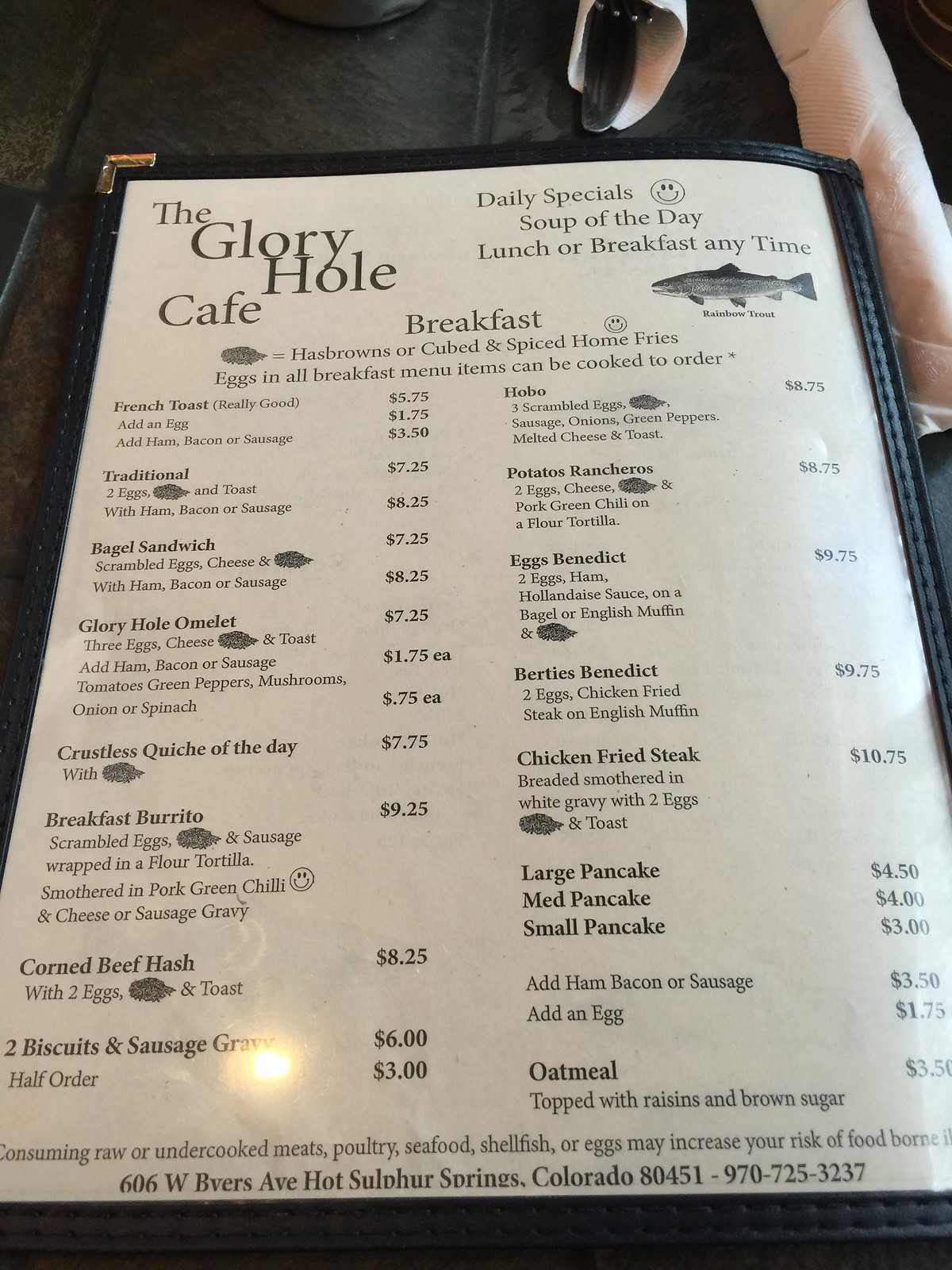Certainly! Here’s a detailed and cleaned-up caption for the picture of the menu:

---

The image showcases a detailed menu from The Glory Hole Cafe, encased in a protective plastic cover with black edges, likely placed on a table. At the top left, the menu lists "The Glory Hole Cafe" alongside cheerful daily specials, highlighted by a smiley face. The specials include a "Soup of the Day" and the enticing option of "Lunch or Breakfast Anytime."

Below this, a vivid illustration of a rainbow trout is accompanied by the text "Rainbow Trout."

Centrally, at the top, the breakfast section offers a variety of dishes such as hashbrowns or cubed and spiced home fries, emphasizing eggs and customizable breakfast items.

The menu then splits into two sections:

**Left Section:**
- **French Toast**: Described as "really good" for $5.75. Add an egg for $1.75 or ham, bacon, or sausage for $3.50.
- **Traditional Eggs and Toast**: Served with ham, bacon, or sausage for $8.25.
- **Bagel Sandwich**: Priced at $7.25, featuring scrambled eggs, cheese, and a choice of ham, bacon, or sausage for $8.25.
- **Glory Hole Omelet**: A three-egg omelet with cheese and toast for $7.25. Optional add-ins like ham, bacon, sausage, tomatoes, green peppers, mushrooms, onions, or spinach for an additional $1.75 each.
- **Crustless Quiche of the Day**: Offered at $7.75, accompanied by a small, indistinct drawing.
- **Breakfast Burrito**: Includes scrambled eggs, a small, unidentifiable item, and sausage wrapped in a flour tortilla for $9.25. Options to smother in pork green chilies, cheese, or sausage gravy.
- **Corned Beef Hash**: Priced at $8.25, served with two eggs, potatoes, and toast.
- **Two Biscuits and Sausage with Gravy**: Available for $6.00, with a half-order priced at $3.00.

**Right Section:**
- **Hobo Special**: At $8.75, consists of three scrambled eggs, potatoes, sausage, onions, green peppers, melted cheese, and toast.
- **Potato Rancheros**: Two eggs, cheese, potatoes, and pork green chilies on a flour tortilla for $8.75.
- **Eggs Benedict**: Two eggs, ham, and hollandaise sauce on a bagel or English muffin for $9.75.
- **Birdie's Benedict**: Priced at $9.75, featuring two eggs and chicken fried steak on an English muffin.
- **Chicken Fried Steak**: At $10.75, breaded and smothered in white gravy, served with two eggs, potatoes, and toast.
- **Pancakes**: Available in large ($4.50), medium ($4.00), and small ($3.00) sizes. Add ham, bacon, or sausage for $3.50 and an egg for $1.75.
- **Oatmeal**: Topped with raisins and brown sugar for $3.50.

At the bottom of the menu, a health advisory warns that consuming raw or undercooked meats, poultry, seafood, shellfish, or eggs may increase the risk of foodborne illness. 

The cafe's address and contact details are listed: 606 West Beaver Avenue, Hot Sulfur Springs, Colorado 80451. Phone number: (970) 725-3237.

The menu is aesthetically simple, rendered in black text on an off-white background.

---